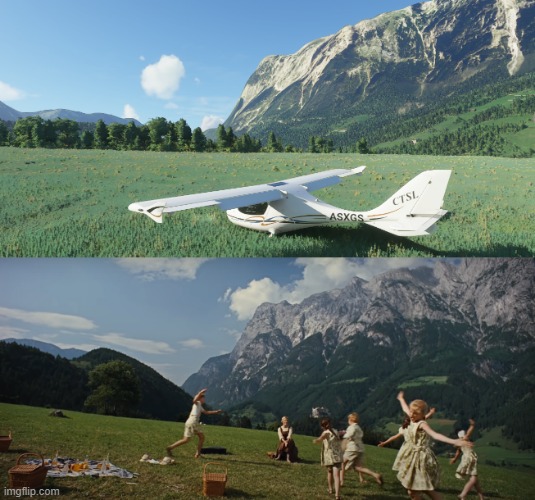The image consists of two distinct photographs arranged one above the other. The top photograph features a sprawling grassy field, upon which a large helicopter, resembling a private aircraft, is prominently displayed. This helicopter is equipped with a sizable white propeller at its top, and it appears capable of accommodating around four passengers, akin to the capacity of a private jet. The aircraft is adorned with black lettering on its side reading "A-S-X-O-S," and additional markings on its tail section that seem to spell out "C-T-S-L" or a similar abbreviation. In the background of the top image, a massive stone wall runs diagonally, adding a unique visual element to the scene. Dotted with a few trees, the landscape is bathed in clear skies, punctuated only by small patches of clouds.

The bottom photograph captures a scene later in the day, evident from its darker tones. It depicts a similar grassy field, but instead of an aircraft, there are several children engaged in playful activities. The presence of various equipment and picnic materials in the bottom left corner suggests a recreational atmosphere. The overall environment in both images shares a pastoral quality, yet each reflects a different time of day and focal activity.